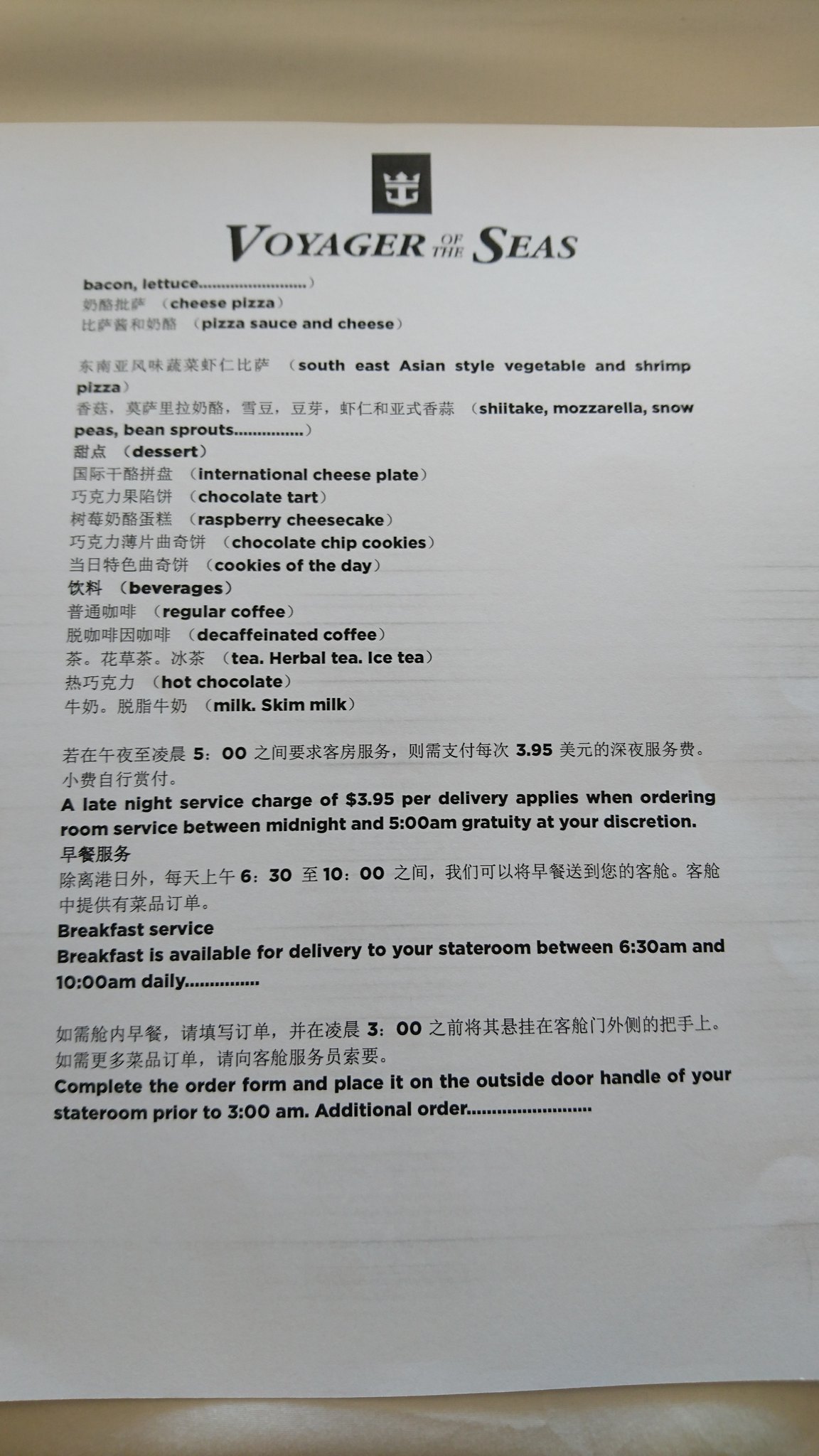A photograph of a receipt from Voyager of the Seas, laid atop a brown wooden surface. The receipt, printed on white paper, displays the ship's logo—a black square featuring two horizontal lines with intricate details on either side. The top section of the receipt lists a diverse breakfast menu, including options such as bacon, lettuce, cheese pizza, pizza with sauce and cheese, Southeast Asian style vegetable shrimp pizza, international cheese plate, chocolate tart, raspberry cheesecake, chocolate chip cookies, and the cookie of the day. Beverage selections include regular coffee, decaffeinated coffee, tea, herbal tea, iced tea, hot chocolate, milk, and skim milk. The receipt details a late night service charge of $3.95 per delivery for room service orders between midnight and 5 a.m., with gratuity left to the guest's discretion. The breakfast delivery service is available to staterooms from 6:30 to 10:00 a.m. This information is also translated into Chinese, with each line item accompanied by its corresponding translation.